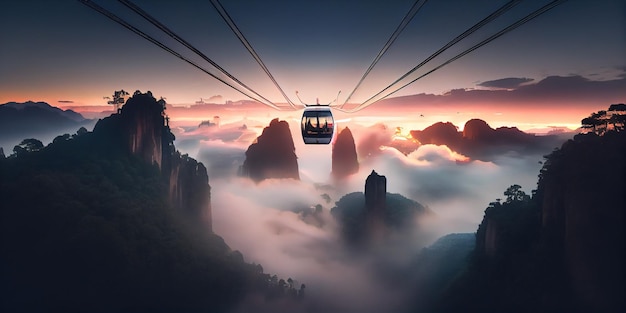The image depicts a mystical and magical scene, possibly AI-generated, featuring a gondola-style cable car suspended high in the sky. The gondola, centrally positioned and enclosed with a compartment section that appears to accommodate two passengers, is tethered to cables that stretch horizontally across the image. The sky above showcases a dramatic gradient, transitioning from a dark navy blue at the top to a vibrant pastel of pink and yellow near the horizon, suggesting a sunrise or sunset. Below this ethereal sky, thick white clouds, tinted with pink and yellow hues, envelop the scene, further enhancing the dreamlike atmosphere. Poking through these clouds are the jagged tips of picturesque mountains, some adorned with lush green vegetation. The entire composition conveys a sense of serene elevation and wonder, as the gondola glides effortlessly above the mountainous terrain and through the misty, illuminated clouds.